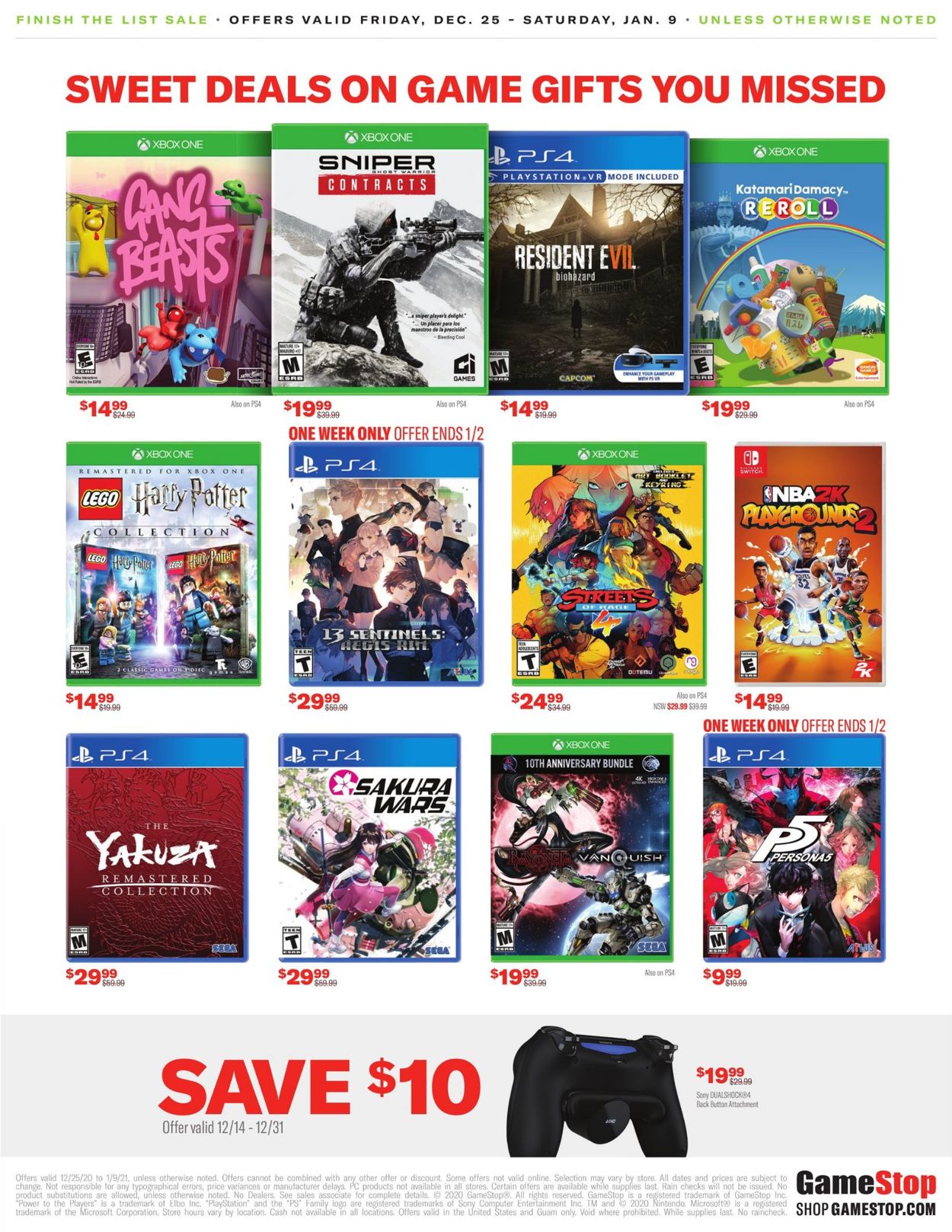**GameStop.com Finish the List Sale**

At the very top of the image, vibrant green text announces the "Finish the List Sale." Just below this, in black text, it states, "Offers valid Friday, December 25th to Saturday, January 9th. Unless otherwise noted," with "unless otherwise noted" in green for emphasis. Beneath this is a bold red banner proclaiming, "Deals on Gifts You Missed."

The image features a meticulously organized list of games for Xbox One and PS4. The most prominent game, highlighted in green, is for Xbox One titled "Sniper's Contract." The game is depicted with an image of a person holding a sniper rifle, rendered in striking black and white contrast. Below this image, the price is prominently displayed as $19.99.